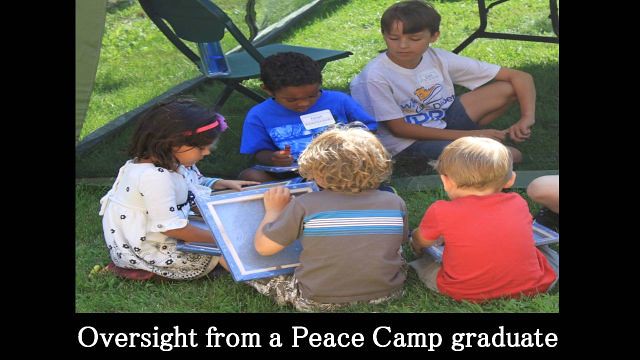This horizontally oriented rectangular photograph depicts five children sitting in a circle on a lawn, engrossed in activities involving blue poster boards. The scene appears to be from an earlier time, possibly the 2000s, evident by the children's styles. Sunshine filters through, casting shadows and suggesting an outdoor setting perhaps featuring a pop-up tent, black chairs, and a folding table visible in the background.

The image is bordered on the left, right, and bottom with a thick black border. At the bottom, written in white font, are the words, "Oversight from a Peace Camp Graduate."

In the image, two boys are seated toward the back; one in a blue t-shirt with a white rectangular name tag, and the other in a white t-shirt with a similar name tag. A little girl in a white dress is positioned to the left side of the photo, viewed from the side. In the front, facing away from the camera, are two more boys: one in a gray shirt with blue and white stripes, and another in a red t-shirt. All the children are looking down at the objects they are holding, deeply engaged in their shared activity.